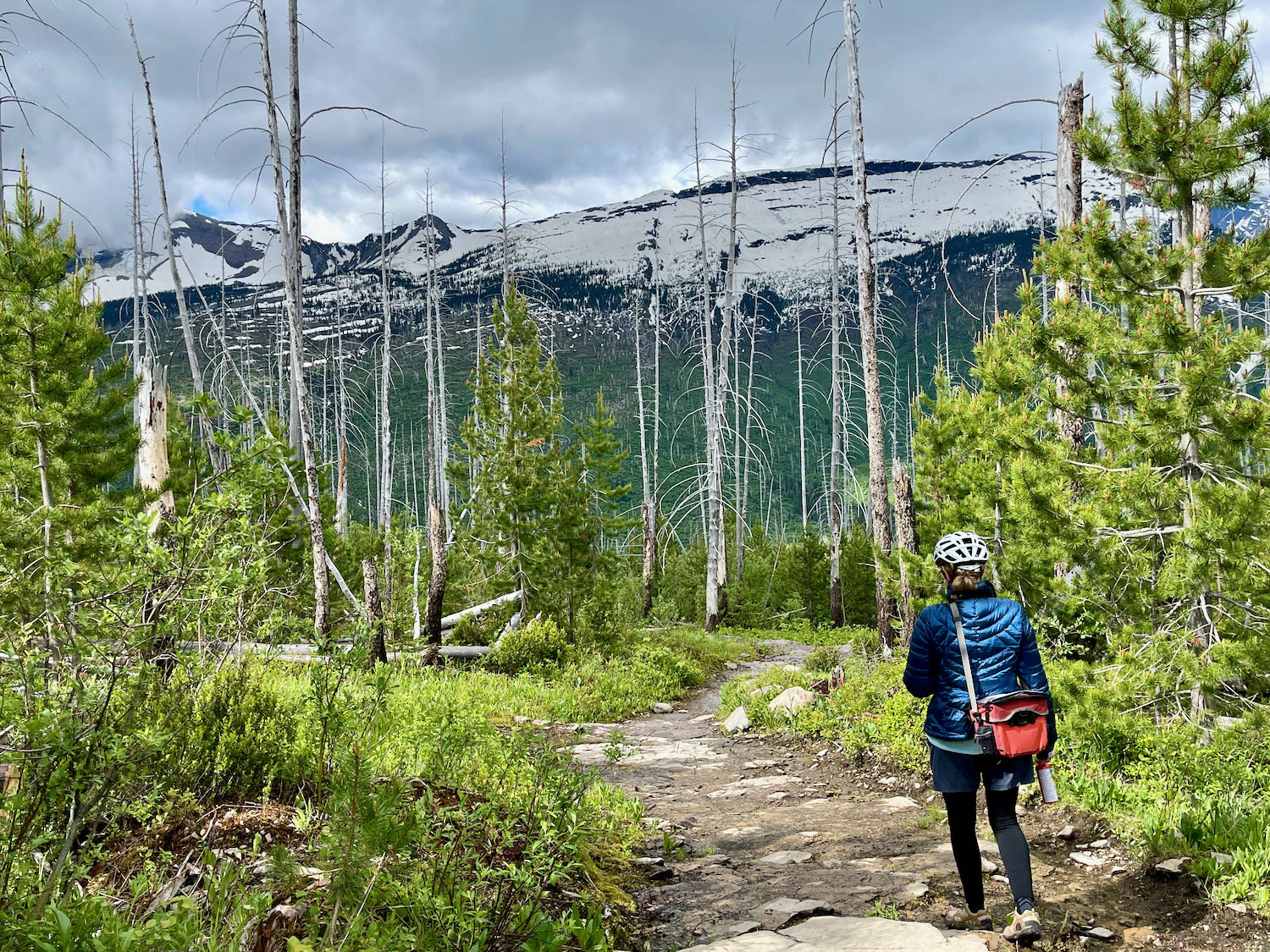This color photograph, taken in landscape orientation at Glacier National Park, captures the back view of a woman hiking along a rugged dirt pathway. She is dressed in a navy blue puffer jacket and black leggings, with a white bicycle helmet on her head. A red backpack is draped over her right shoulder, and she holds a bottle in her right hand. As she walks on the trail, which is scattered with flat, gray stones, she navigates through a diverse landscape featuring live pine trees and grassy patches on both sides, interspersed with bare, skinny tree trunks. In the distance, a majestic mountain range looms, its lower half lush and green, while the upper half is jagged and snow-covered. The scene is set under an overcast, gray sky, adding to the dramatic atmosphere of this realistic representation of hiking in the great outdoors.